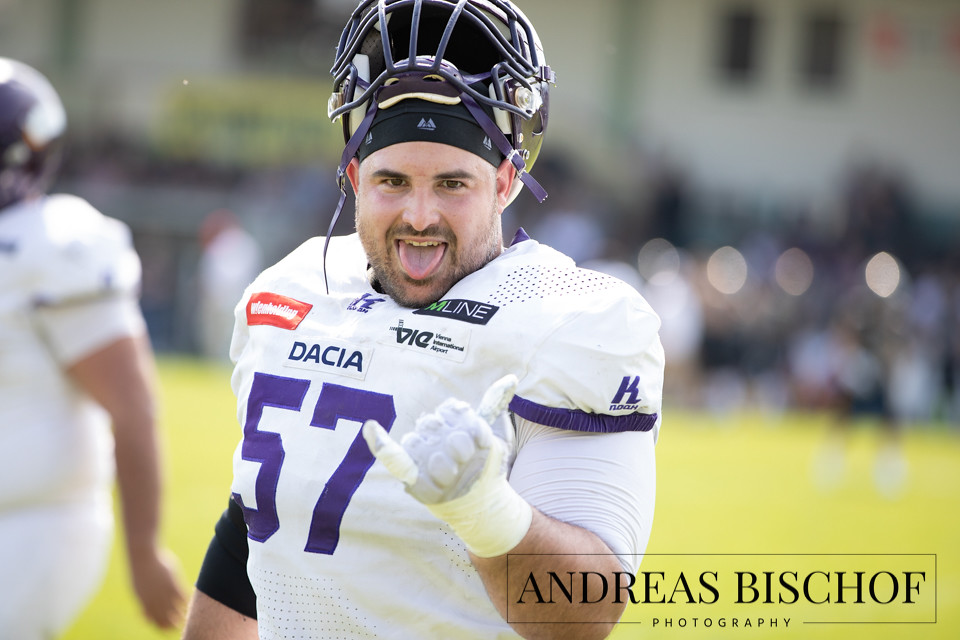The photograph, captured by Andreas Bischoff Photography, features a close-up of a jubilant Caucasian football player with light-colored skin. He is situated outdoors on a blurred green field, surrounded by other indistinguishable players and fans. The athlete sports a heavily padded football jersey, primarily white with dark purple accents and the number 57 visible. Though he wears a black helmet, it is perched atop his head, revealing his dark brown eyes, bushy dark brown eyebrows, and a complementing dark brown mustache along with a 5 o'clock shadow beard. Beneath his helmet, a black headband wraps around his forehead. Adding to his spirited demeanor, he is making the "Hang Ten" sign with one hand—thumb and pinky extended—while his tongue playfully sticks out, showcasing yellow teeth.